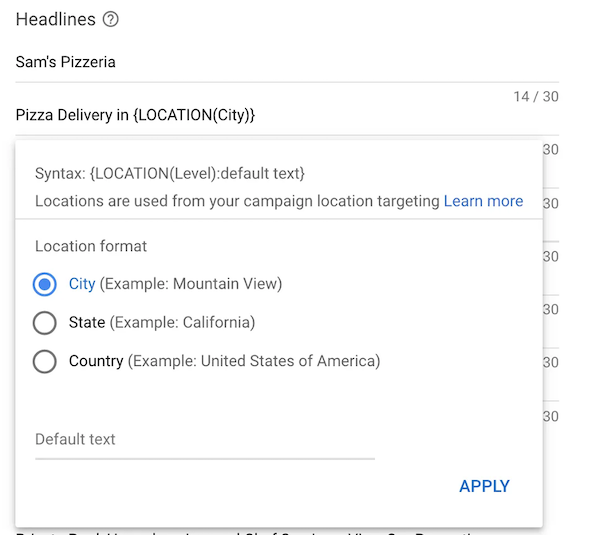At the top left corner of the image is the word "Headlines," followed by a question mark inside a circle. Directly below this, "Sam's Pizzeria" is written, with a long horizontal line extending to the right. Next is the text "Pizza Delivery Inn" enclosed in parentheses with the words "location" and "city" beside it.

Below this, in gray text, "Syntax: (location, level, default text)" is displayed, followed by another gray text line that reads "locations are used from your campaign location targeting." Additionally, there is an option to click and learn more, presented in blue text.

Below this, there is the text "Location Format" in gray, followed by the word "city" in blue. Adjacent to this, towards the left, is a blue circle filled in, alongside the example text "(example: Mountain View)." Underneath, a white circle (unfilled) is highlighted with the word "state" and the example "(example: California)" in parentheses. Finally, below this, there is another unfilled white circle with the word "country" and the example "(example: United States of America)" in parentheses.

At the very bottom, the term "default text" is written with a long horizontal line underneath, and in the bottom right corner, the word "apply" is displayed in blue text.